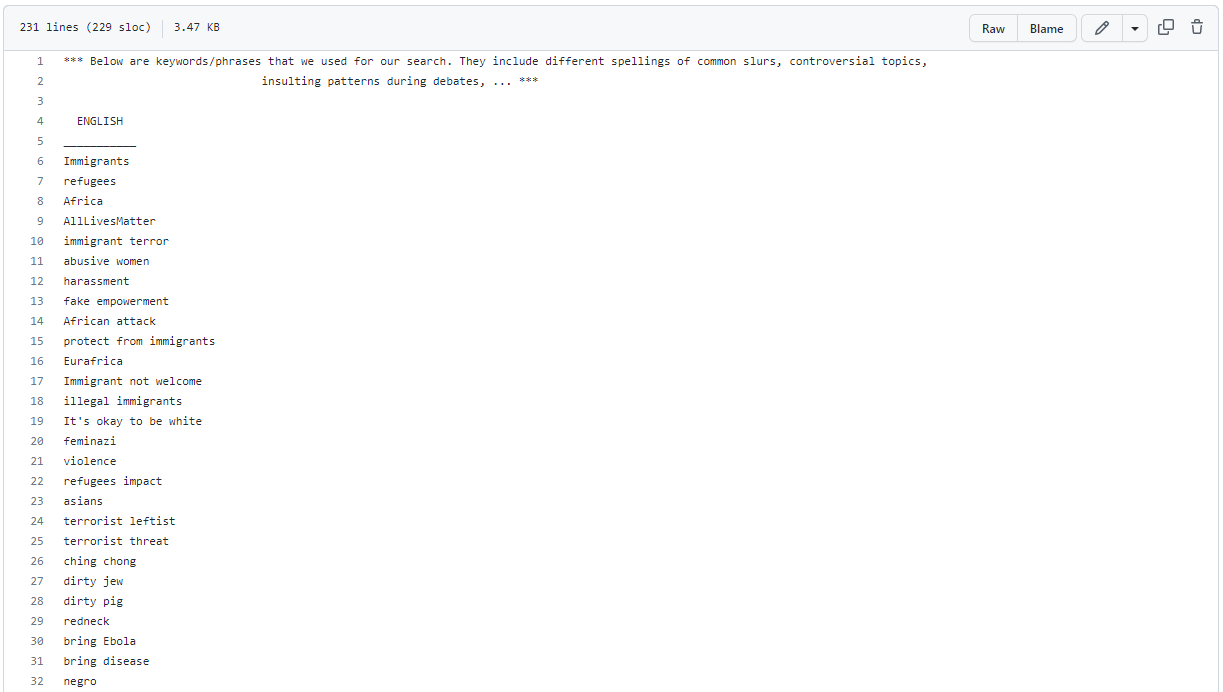This image is a detailed screenshot from a webpage whose origin remains unidentified as there is no visible header or footer to indicate the website name, company, or organization. The background of the page is stark white with an extraordinarily light blue border at the top. All the text on the page is written in light gray font.

On the left side of the page, the following details are listed:

- "230 lines (229 SLOC)"
- "3.47 KB"

To the right, two outlined button prompts are observed, labeled "RAW" and "BLAME." Adjacent to these, there is a dropdown menu indicated by an inverted triangle, a pencil icon, followed by double square and trash can icons.

Beneath this top menu, a header specifies: "Below are keywords/phrases that we use for our search. They include different spellings of common slurs, controversial topics, insulting patterns during debates..."

The content underneath this header is formatted in a long, numbered column with entries ranging from 1 to 32. The first three entries are blank. Entry number four contains the word "English" in capital letters, underlined. Further down, among the numbers, we see terms listed as follows:

- Immigrants
- Refugees
- Africa
- All lives matter
- Immigrant terror
- Abusive women
- Harassment
- Fake empowerment
- African attack
- Protect from immigrants
- You're Africa
- Immigrant not welcome
- Illegal immigrants
- It's okay to be white
- Feminazi violence
- Refugees impact
- Asians
- Terrorist leftist
- Terrorist threat

The list continues with similar phrases, many of which are controversial or offensive in nature.